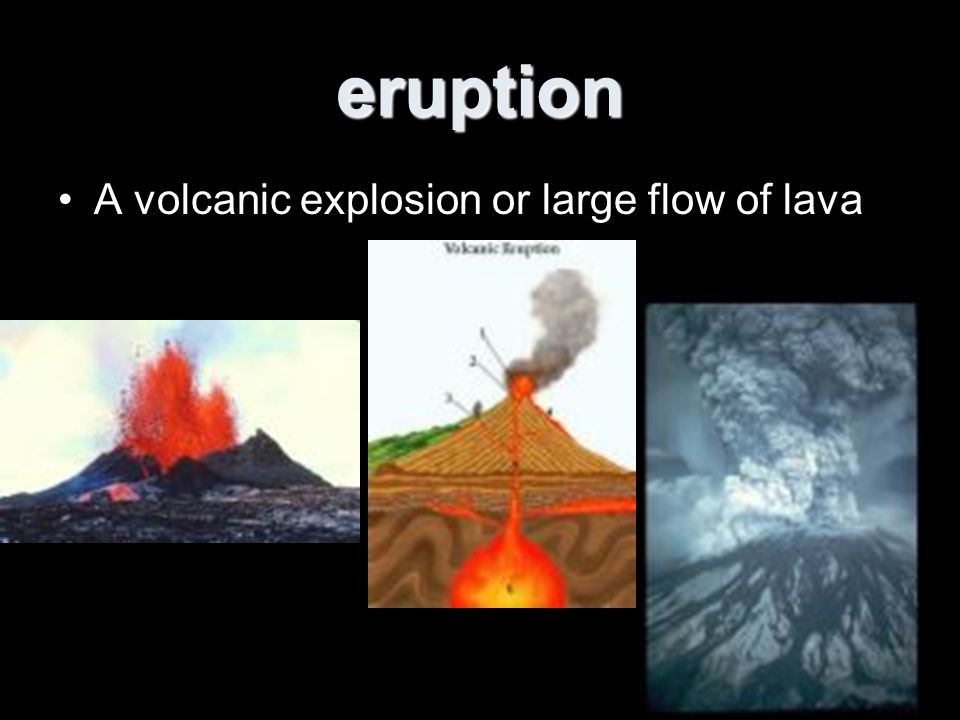The slide, designed in a black background with white text, features the title "eruption" at the top, followed by a bullet point description, "a volcanic explosion or large flow of lava." The slide showcases three distinct images in a row at the bottom. 

The leftmost image depicts a dark, gray mountain or hill, with vibrant red-orange lava erupting dramatically into the sky. The scene includes a small structure with a red roof in the foreground, possibly a house or barn. The contrast between the dark mountain and the fiery eruption is striking, with a backdrop of smoky white.

The central image appears to be a digital diagram of a volcanic eruption. It includes a labeled illustration, possibly reading "Volcanic eruption." This diagram shows a cross-section of a volcano with red-orange fire emanating from below the ground, illustrating the underground lava channels extending laterally and vertically through the soil to the surface. Behind the volcano, there's a green hillside, making the smoke plume and eruption details more prominent against the white sky background.

The rightmost image portrays another volcanic eruption but with a darker, more subdued aesthetic. The entirety of the image is in shades of gray, illustrating ash and smoke billowing from the erupting volcano. This image also hints at the underground activity, resembling tree branch-like patterns above and below the ground.

Overall, the slide seems like part of a PowerPoint presentation, using a combination of realistic imagery and informative diagrams to convey the dramatic and complex nature of volcanic eruptions.